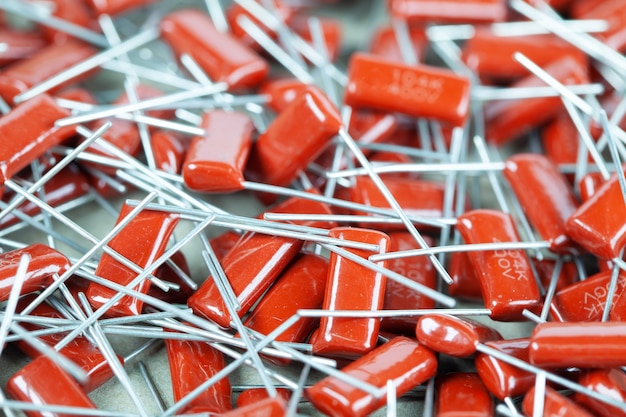The image features a large pile of red rectangular objects, each affixed with a metallic pole or stick emerging from one side. These red rectangles, possibly made of resin or plastic, have a shiny surface and seem to be intricately manufactured. The metal poles are stacked haphazardly atop one another, contributing to a chaotic assembly of these red objects on what appears to be a gray surface. A closer inspection reveals that there is some text on the red rectangles, with the number '4K' vaguely discernible among the writings. The overall scene presents a scattered, unique arrangement of these synthesized items, which evoke curious speculation about their exact purpose or function.